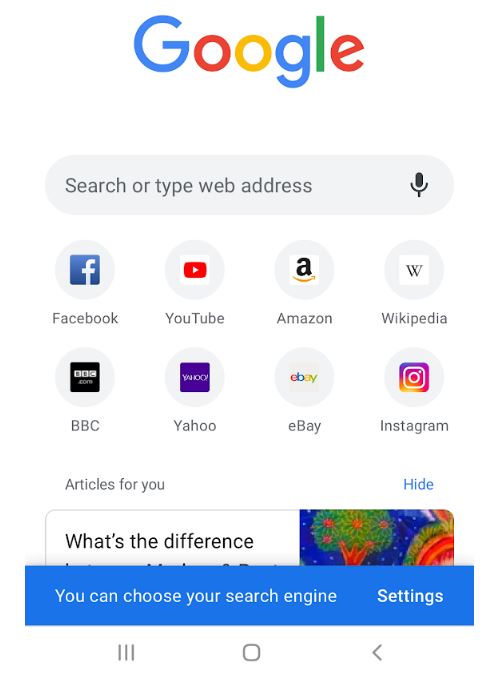A browser screen is depicted displaying the Google homepage. The distinct Google logo includes a blue 'G', a red 'o' encased in a circle, a yellow 'o' also in a circle, another lowercase blue 'g', a green 'l', and a red 'e'. Below the logo is a search bar with a microphone icon to the right. The search bar is a gray rectangle. 

Beneath the search bar, a selection of app icons is displayed, featuring familiar options such as Facebook, YouTube, Amazon, Wikipedia, BBC, Yahoo, eBay, and Instagram. Below these icons is a gray section labeled "Articles for you" with blue text to the right reading “Hide.” Adjacent to this, there is a small image accompanied by the text "What's the difference," written in black.

Moreover, a horizontal blue bar crosses the screen containing the text "You can choose your search engine," with a "Settings" label to its right. Further down, an image features a tree bearing what appear to be apples, set against a blue background. There is also a small green and red bush. At the bottom, navigation icons are displayed: a left-pointing triangle, a central square, and three vertical lines to the left. The entirety of this layout is set against a white background.